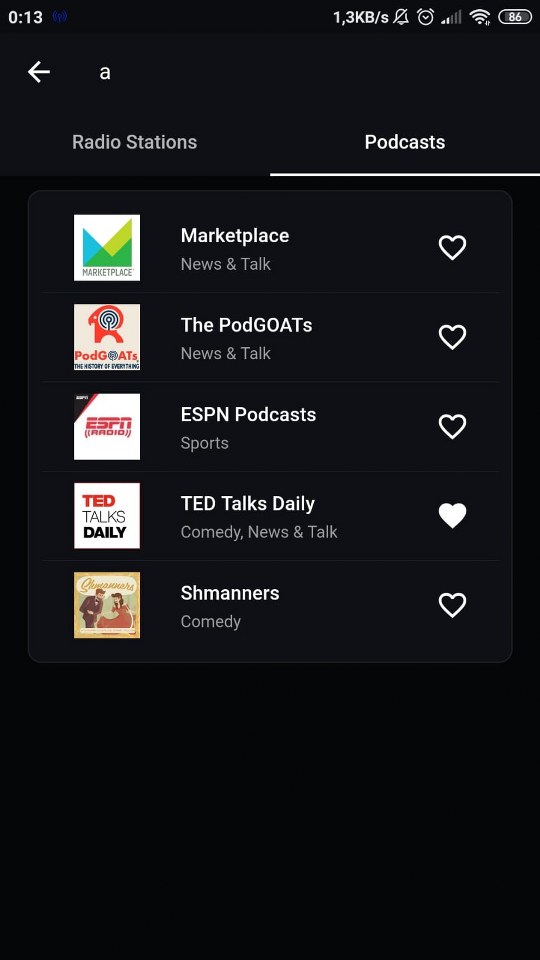This image showcases a website with a predominantly black background. At the top, the time is displayed as "01:13", accompanied by various icons and metrics on the right, including "1.3 kb/s" for data speed, a muted bell icon, an alarm clock icon, two signal bars, and battery life at "86%". All these elements are depicted in white.

On the left-hand side of the screen, a left-pointing arrow is accompanied by a small white letter "A". Beneath this, there are navigational labels with "Radio Stations" and "Podcast". The "Podcast" label is underlined with a white line, indicating it is the currently selected category.

Below the navigation labels, categories for podcasts are listed in white text, starting with "Marketplace". This entry features a white box displaying various shades of green and blue lines, and it reads "Marketplace" followed by "News and Talk" with an outlined heart icon next to it.

Next is "POD Goats", where "GOATS" is capitalized. This entry has a white box with what appears to be a red 'R' or an animal shape, alongside a black and white bullseye circle. The caption reads "Pod Goats, the 45th Story of Everything" with a white heart to the right.

Following that is "ESPN Podcast", categorized under "Sports". It includes a white box and a red "ESPN Radio" logo in the middle. Like all entries, this one also features a white heart icon to the right.

The subsequent entry is "TED Talks Daily", listed under "Comedy News and Talk". It includes a white box with the letters "TED" in red and "Talks" in black, followed by "Daily" in thick black letters. The heart icon next to this entry is filled in, likely indicating it is the selected choice.

The final podcast entry is titled "SHMANERS" under the "Comedy" category. It features a yellow box with the label "Shmaners" and cartoonish characters of a man and a woman next to it. This entry also has an unfilled white heart icon to the right.